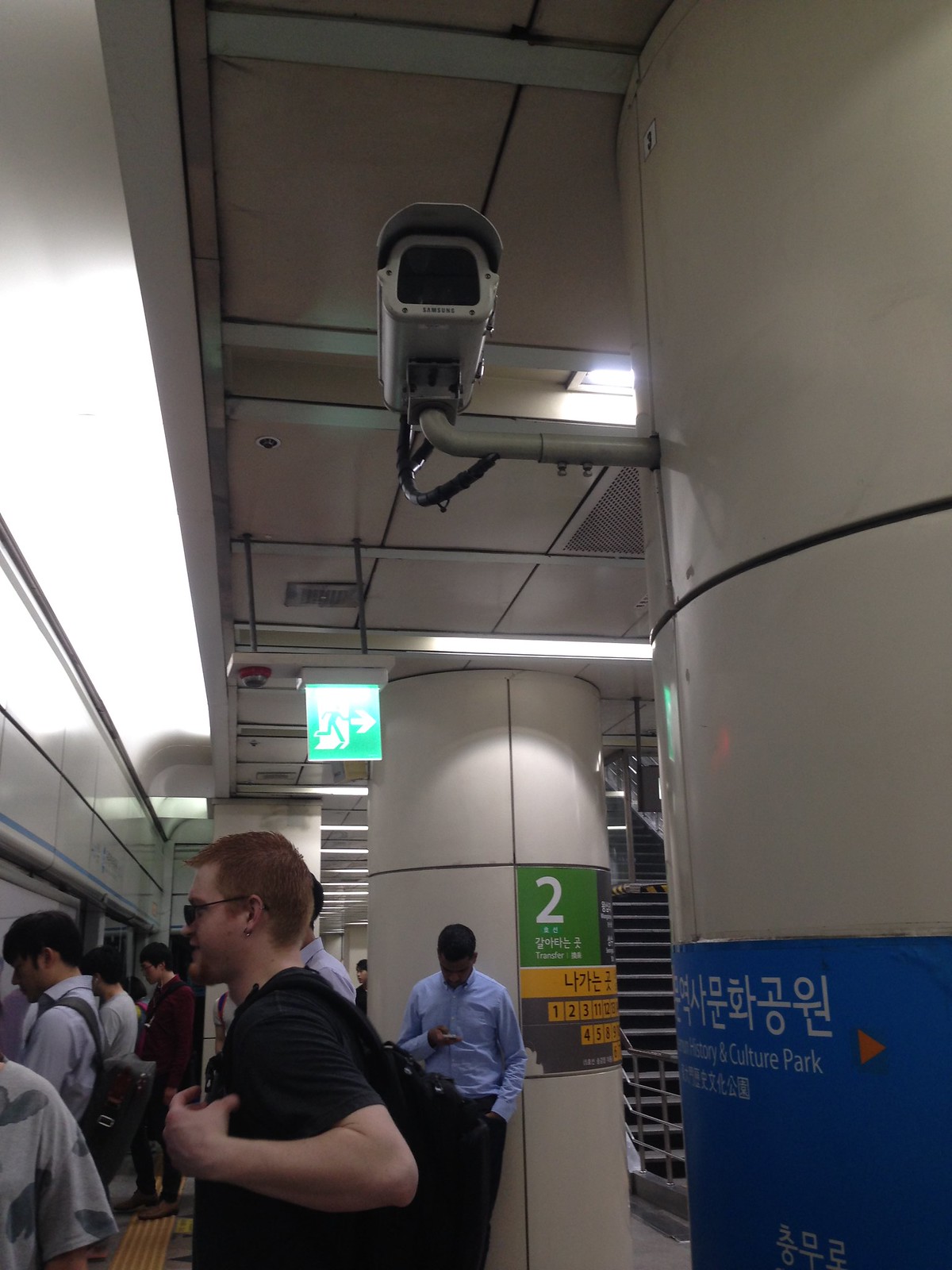This photograph captures a bustling indoor scene, likely within a Korean metro or subway station, evident from the signage in Korean characters. The station boasts a modern infrastructure, characterized by its large, cylindrical pillars, white-tiled ceilings, and installed CCTV cameras. An array of signs are visible, including a blue sign on one pillar reading "History and Culture Park" with an orange arrow pointing right, and another green sign with a white number 2 on the central pillar, supplemented by additional signs with Asian characters and arrows indicating directions.

People are queued at various ticket counters, awaiting their turn. The man closest to the camera has short, brownish-red hair, wears sunglasses, a black t-shirt, and carries a black backpack, holding its strap with his left arm. Not far behind him, a man in a light blue shirt leans against the central pillar, engrossed in his mobile phone. Additional details include visible smoke detectors, lights, and staircases that add to the station's busy ambiance. Despite the lack of visible trains, the scene effectively captures the essence of a bustling subway environment, with everyone uniformly facing towards what might be an approaching train or the ticket counters.